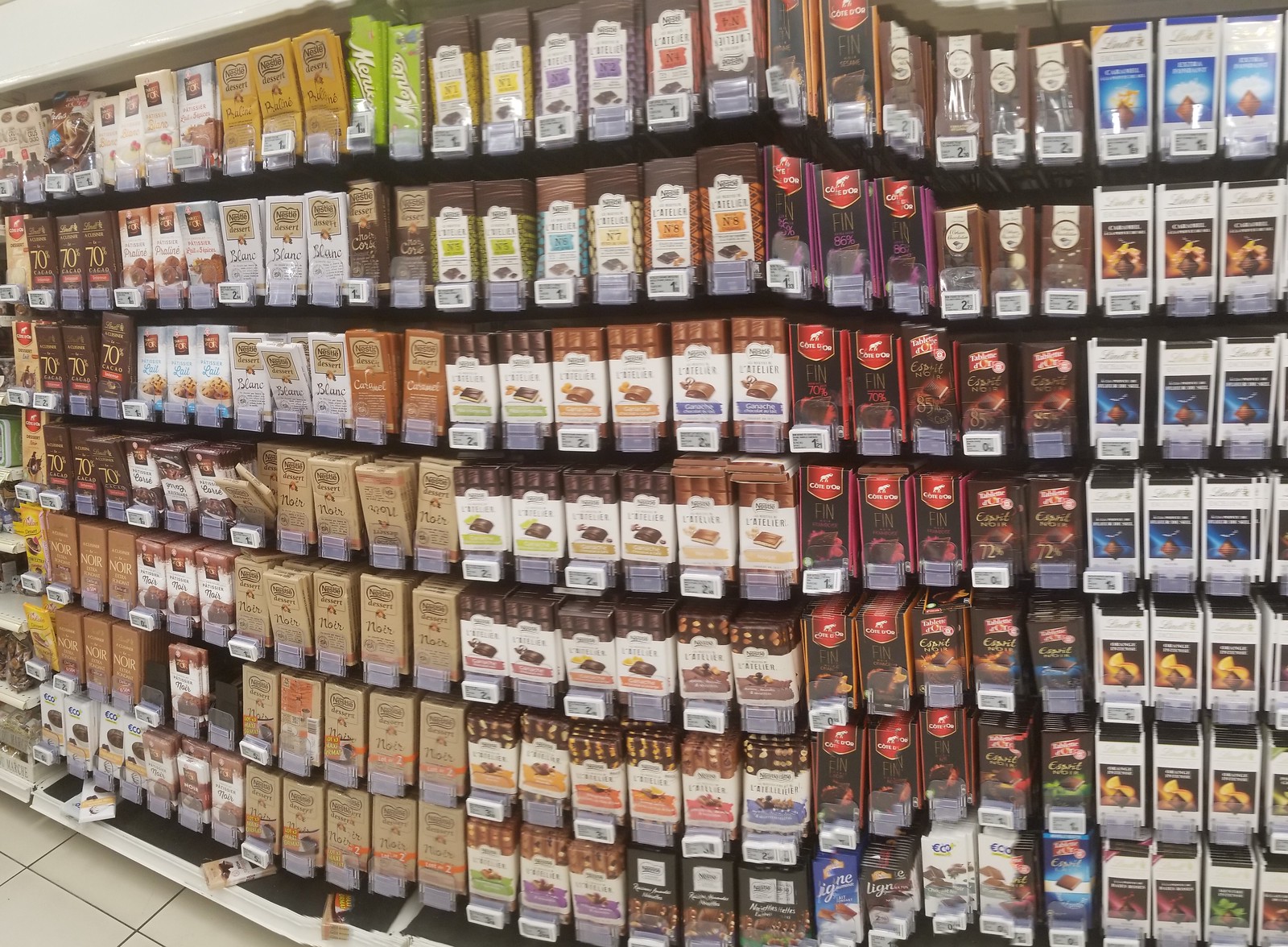The image captures the interior of a well-stocked store. In the bottom left corner, a pristine white tile floor is visible. The image primarily showcases rows of shelves packed with neatly arranged products, displayed lengthwise. The products, which appear to be fine chocolate bars, are organized with precision. The packaging varies, featuring tan, brown with red writing, white, and multi-colored wrappers. Each chocolate bar is placed snugly next to its neighbor, creating an impression of abundance. The shelves are densely packed, with the front edges displaying the colorful wrappers prominently. The shelves extend upwards, nearly reaching the ceiling, with a sliver of white ceiling visible at the top of the photograph. The overall scene is one of a well-organized retail space brimming with delectable chocolate offerings.